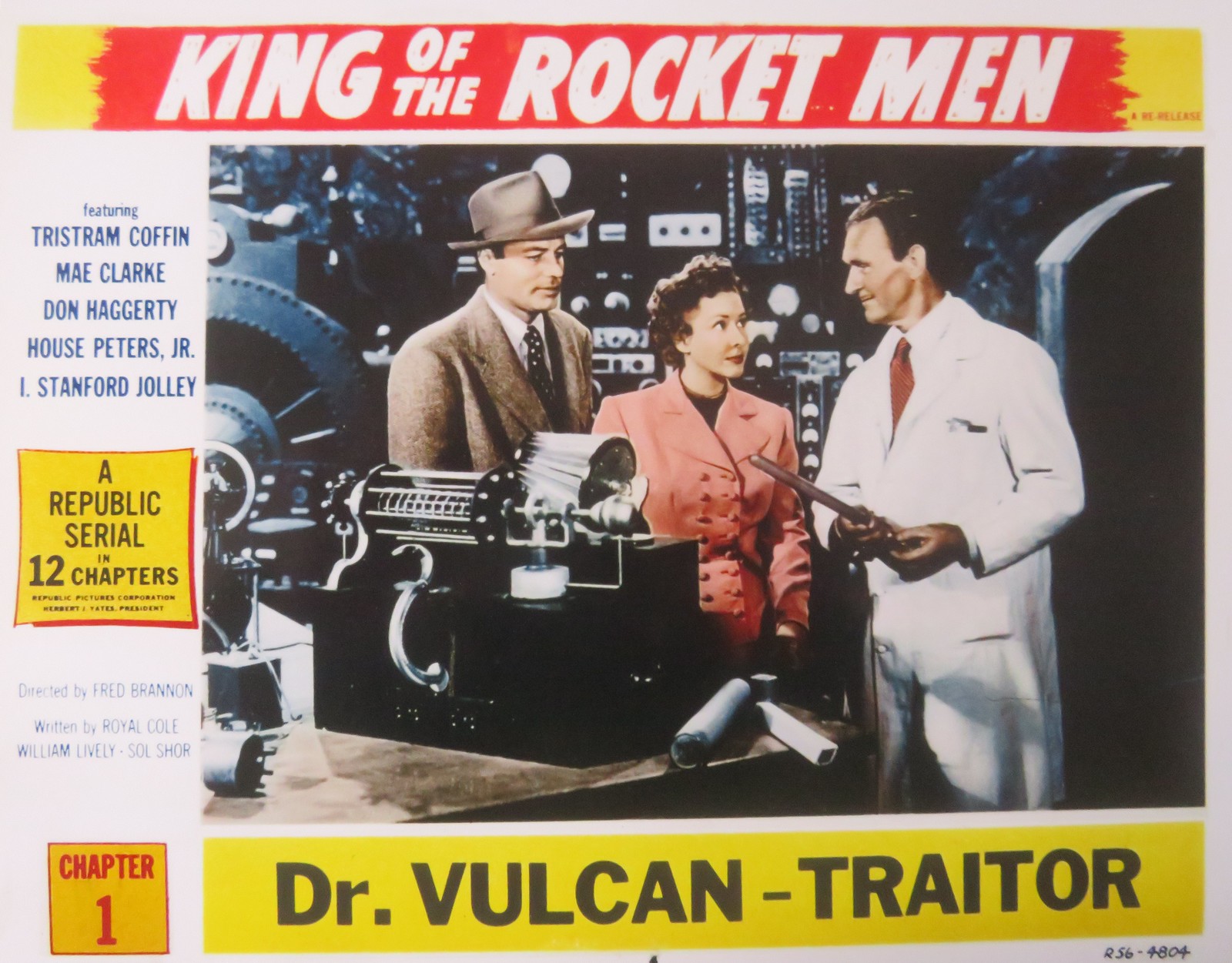This rectangular image, wider than it is tall, features a prominent light gray background with a vivid, multicolored banner stretching from left to right at the top. The banner starts with yellow at the left tip, transitions to red in the center where the bold white text reads "King of the Rocket Men," and then shifts back to yellow at the right tip. Below this, on the left-hand side, is a blue text listing the main actors: "featuring Tristam Coffin, May Clark, Don Haggerty, House Peters, Jr., and L. Stanford Jolly." Adjacent to this is a yellow square with black print stating, "a Republic serial in 12 chapters." Further down, light blue text credits the director and writers: "directed by Fred Bannon, written by Royal Cole, William Lively, Sol Shore."

In the bottom left-hand corner, within another yellow square edged in red with red text, it reads "Chapter One." On the right, a yellow banner with black text announces, "Dr. Vulcan, Traitor." Above this is an older image featuring two men and a woman surrounded by scientific equipment. One man is in a white uniform, possibly the illustrated doctor, while the scientist's intense gaze meets the curious looks of the man and woman in front of him. In the lower right-hand corner, the letters and numbers "R56-4804" are handwritten.